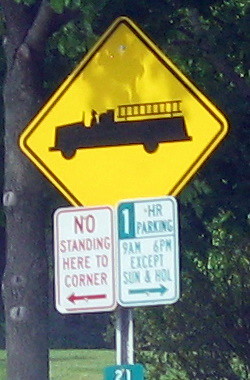The photograph features a yellow sign with a prominent, black fire truck icon, indicating that fire trucks may exit the area at any moment. Directly beneath it, another sign reads "No standing here to the corner," with bold red letters on a white background. Below this directive, there's a white sign with green letters stating "One hour parking, 9 a.m. to 6 p.m. except on Sundays and holidays," accompanied by a green arrow. The background of the image showcases a lush, natural setting dominated by a massive tree trunk on the left, extending upwards beyond the frame. The right side of the photograph is filled with dense bushes, green leaves, and additional trees, creating a shaded, verdant ambiance. Notable details include notches on the large tree where low branches have been cut, and a small green sign displaying the number "21" located at the bottom of the picture.